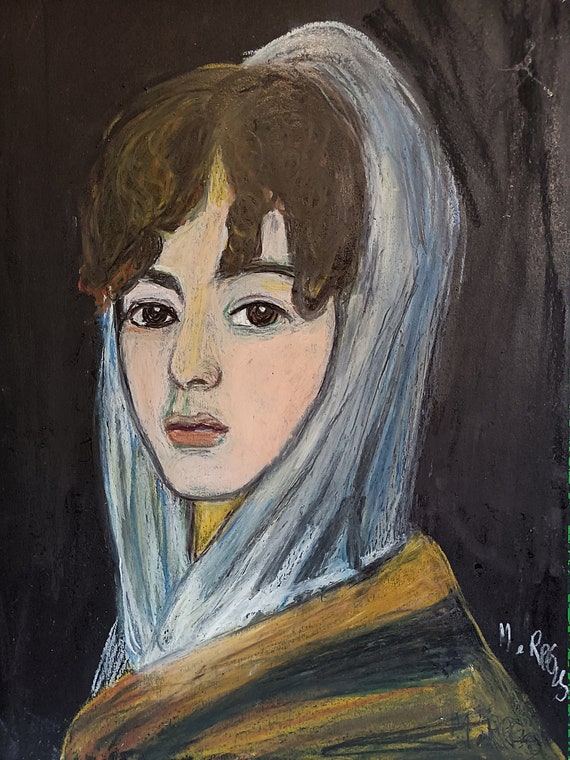This is an image of a painting, possibly created with oil pastels or acrylics, depicting a pale-complexioned young woman with curly dark blonde to golden brown hair. The painting’s black background contrasts starkly with the figure, who is turning slightly to her left but gazes directly at the viewer with brown eyes. Her facial expression appears rather muted, perhaps dull or forlorn. She wears a white or bluish-gray head cover and a yellow and black striped blouse or jacket. The painting features minimal, basic shadowing and lacks strong detail in the hair and gown. A signature in white is visible just above her shoulder, although it's difficult to decipher. Only her head and shoulders are visible in the image.